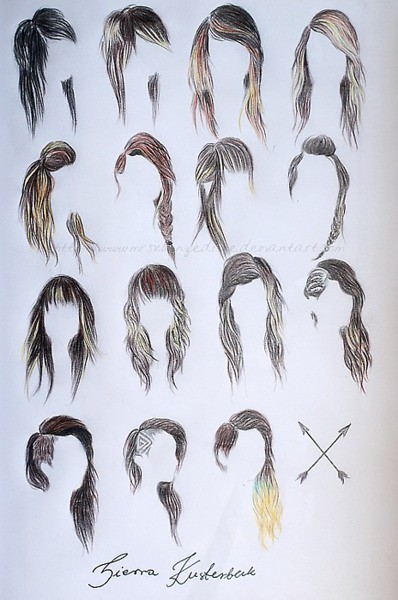This image displays an array of 15 artistically rendered women's hairstyles set against a predominantly white to light gray background. The layout features four rows, with the top three rows containing four hairstyles each, and the bottom row displaying three. Each hairstyle is depicted around white silhouettes representing faces, though no actual facial features or heads are drawn, leaving just the hair illustrated. The hairstyles vary in color from black and brown to some with blonde highlights. In the bottom right corner, where a fourth hairstyle would be, two arrows intersect to form an X. Below the collection, the signature "Sierra Kusterbeck" is inscribed in cursive black text.